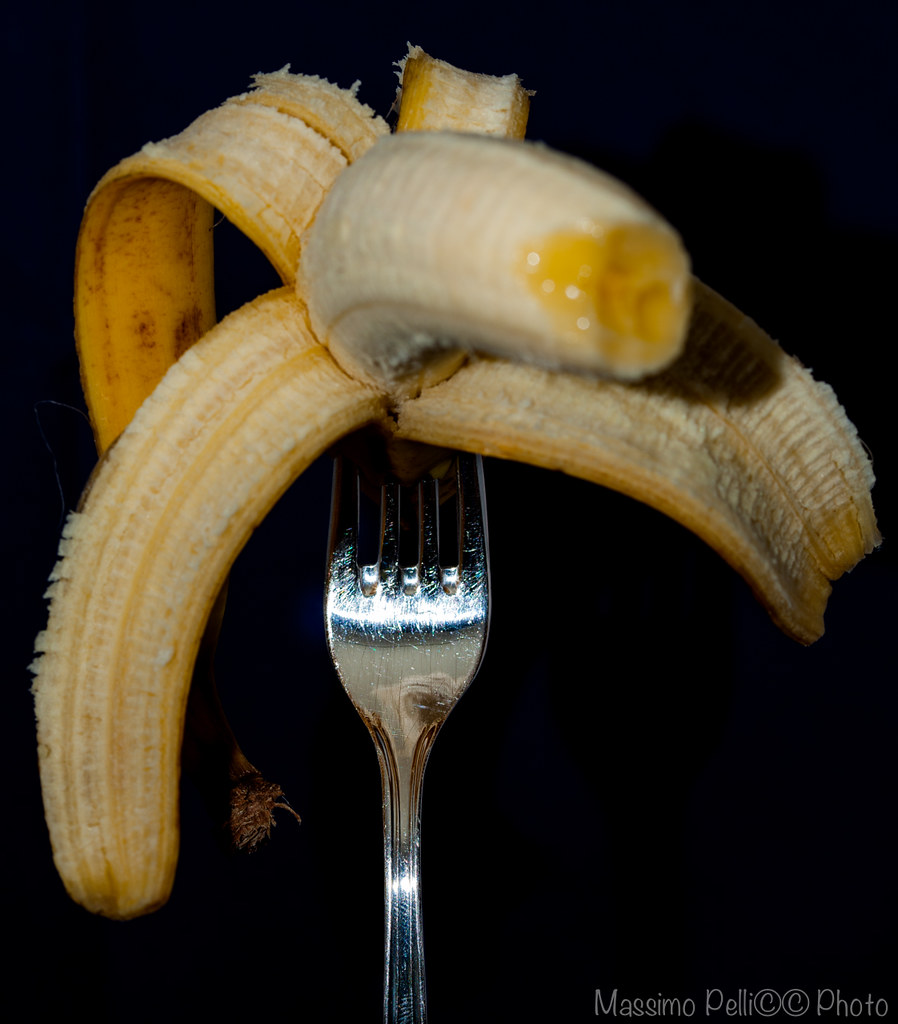In this striking photograph, a banana is prominently displayed, peeled into four delicate sections cascading downwards. The fruit itself is perched atop a fork, though the prongs piercing the banana remain obscured from view. The top tip of the banana, which reveals an eaten section, contrasts sharply against the deep black background with its vibrant yellow hue. At the bottom right corner, the image is marked with the credit "Massimo Pelli © Photo," emphasizing its artistic ownership. An indistinct, husky texture can be observed in the bottom left portion of the image, adding subtle depth to the composition.